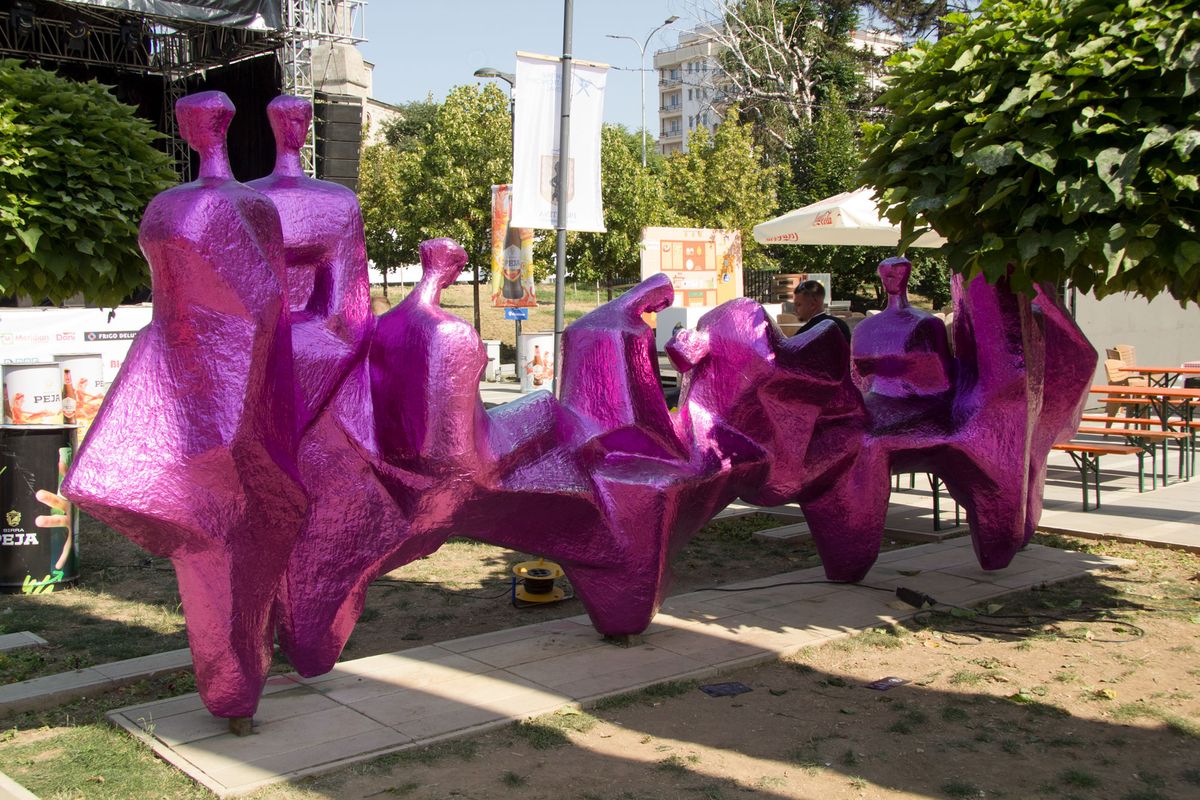This photograph captures a vibrant and intricate modern art sculpture set in an outdoor park-like location. The central focus of the image is a bright pinkish-purple metallic sculpture designed with abstract, angular elements. The figures in the sculpture seem to represent vaguely human shapes engaged in various poses—some standing, others sitting in rows, with each figure connected to the next. In the background, lush trees border the scene, and tall buildings rise above the tree line, giving a sense of being in a city park. To the left, a stage construction is visible, and to the right, there's an arrangement of picnic tables and benches, some with umbrellas. The ground is a mix of dirt and small grass patches, adding a natural texture to the urban setting. The sky above is clear, suggesting a sunny day. Intriguingly detailed, the sculpture features figures with small heads and broad, tapering bases that evoke a cubistic or possibly even a surreal interpretation of people.